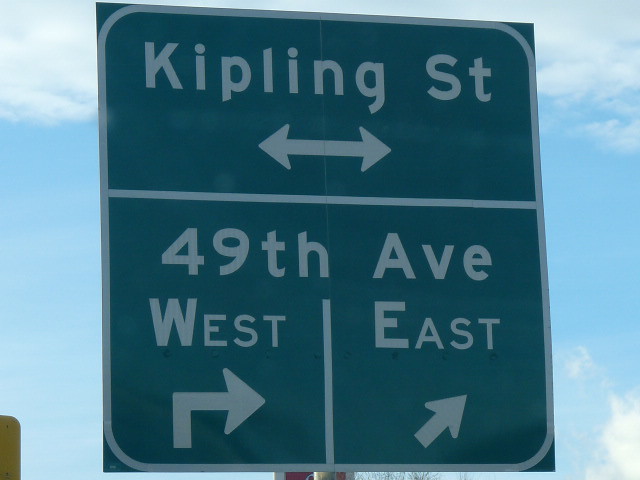This photograph captures a green and white street sign positioned off the side of a highway, set against a picturesque backdrop of a light blue sky adorned with fair weather clouds. The clouds are particularly prominent behind the sign, especially towards the left and right, as well as in the bottom right corner of the image. The top part of the sign reads "Kipling St," with the word "Street" abbreviated. Below this, arrows point both left and right, indicating directions. Further down, the sign displays "49th Ave" with a vertical line running under the "H" in "Ave." To the left of this line, the sign indicates "West" with an arrow pointing right, featuring a distinctive bend. On the right side of the line, it marks "East," accompanied by an arrow that angles up and to the right.